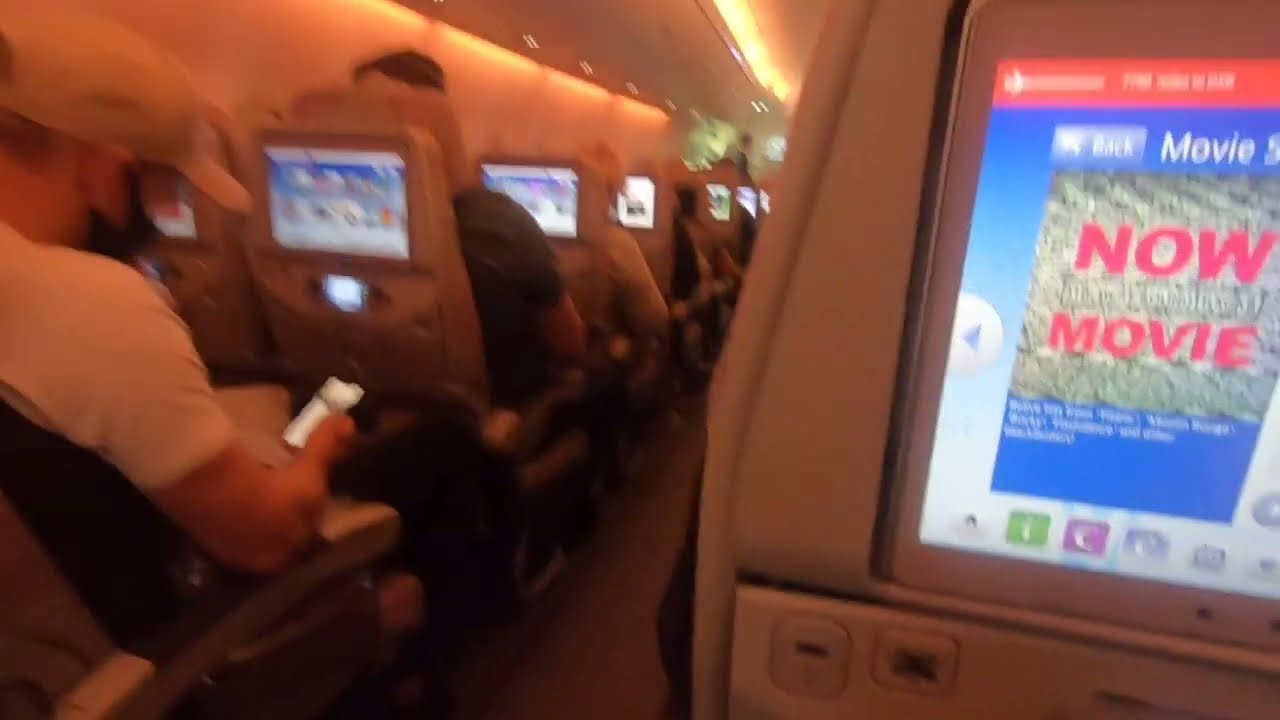The image depicts the interior of a dimly-lit commercial jet, filled with passengers seated on either side of a central aisle. Rows upon rows of seats extend down the walkway, with many passengers engrossed in their cell phones. Notably, a person on the left side of the aisle appears to be texting, while another passenger further down the row is watching a movie. A noticeable detail in the image is a video screen located on the back of one of the seats, displaying the text "Now Movie" in blue, accompanied by control buttons in purple, green, and gray. Among the diverse colors in the image are tones of tan, blue, red, gray, green, purple, and orange. The overall setting unmistakably suggests the interior of an airplane.